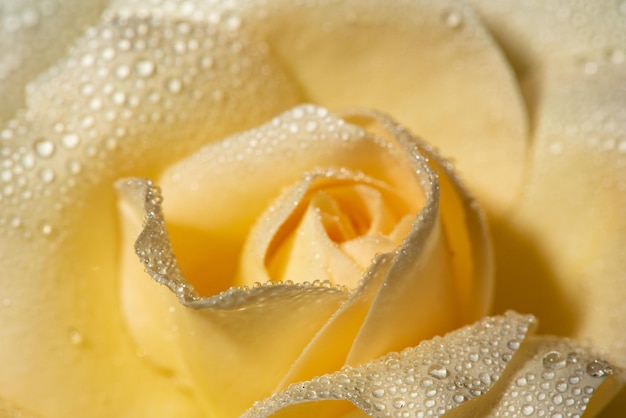The image is a striking close-up photograph of a rose with warm lemony yellow, buttery petals, giving it a visual semblance to vanilla ice cream. The petals are delicately graced with droplets of water, suggesting it has just rained. The center of the rose dominates the image, showcasing both a set of inner petals that have yet to fully bloom and an outer set that is already open, highlighting the intricate patterns and lines where the petals interlock. Tiny filaments or pistils are visible within the flower, adding to the detailed texture. The photograph captures the flower in well-balanced lighting, emphasizing the beads of moisture and the shadows cast by the overlapping petals. The flower occupies the entire frame without any text, confirming it was taken by a real person and not artificially generated. The colors observed are primarily yellow, white, and a hint of orange, enhancing the overall richness of the image.